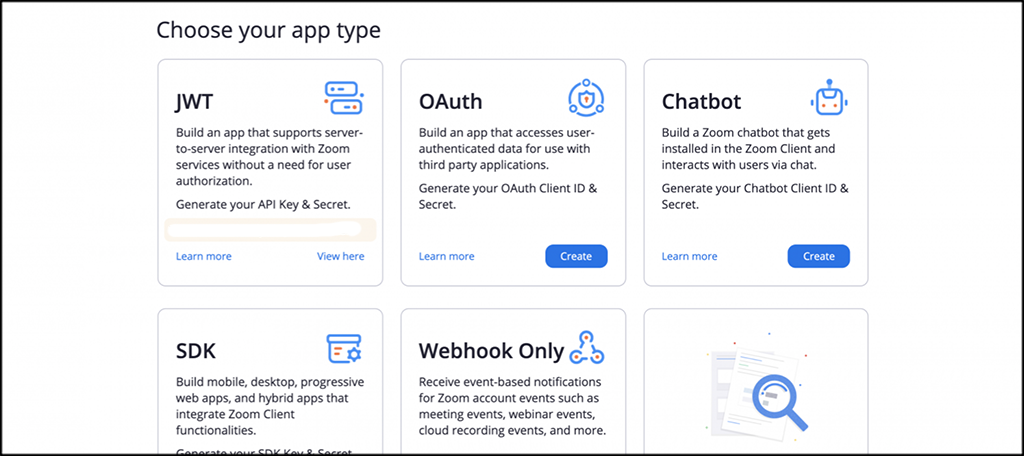**Image Description:**

The image's background is white, and it features the heading "Choose Your App Type" prominently at the top in black text. Below the heading, six options for different application types are presented, each within a distinct section.

1. **JWT (Top Left):**
   - **Icon**: A blue symbol.
   - **Description**: "Build an app that supports server-to-server integration with Zoom service without a need for user authorization. Generate your API Key and Secret."
   - **Buttons**: A "Learn More" button.

2. **OAuth (Top Center):**
   - **Icon**: A blue circular symbol.
   - **Description**: "Build an app that accesses user-authenticated data for use with third-party applications. Generate your OAuth Client ID and Secret."
   - **Buttons**: A "Learn More" button on the bottom left, and a "Create" button on the bottom right.

3. **Chatbot (Top Right):**
   - **Icon**: A blue symbol.
   - **Description**: "Build a Zoom chatbot that gets installed in the Zoom client and interacts with user's chat. Generate your Chatbot Client ID and Secret."
   - **Buttons**: A "Learn More" button and a "Create" button.

4. **SDK (Bottom Left):**
   - **Icon**: A blue symbol.
   - **Description**: "Build mobile, desktop, progressive web apps, and hybrid apps that integrate some client functionalities."

5. **Webhook Only (Bottom Center):**
   - **Icon**: A blue feature spinner.
   - **Description**: "Receive event-based notifications for Zoom account events such as meeting events, webinar events, cloud recording events, and more."

6. **Feature Spinners (Bottom Right):**
   - **Icon**: A blue search symbol.
   
Each option's icon is distinctly blue, maintaining visual consistency across the various sections.